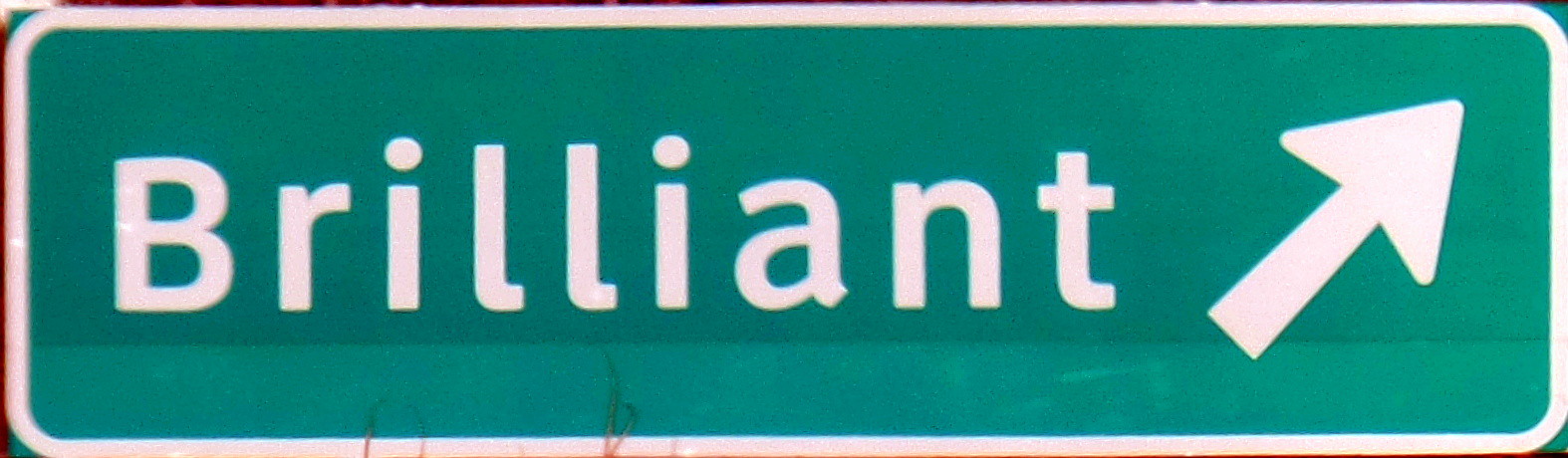The image shows a rectangular, forest emerald green freeway sign with a worn, slightly weathered look, featuring a white border around its edges. In bold, white letters, the sign prominently displays the word “Brilliant,” with the ‘B’ in uppercase and the rest in lowercase. Alongside the text, a white arrow points to the northeast, indicating the exit for "Brilliant." Notably, there are small shrubs growing at the bottom left of the sign, particularly beneath the letters "I" and the second “L.” There is no additional text on the sign, just this striking and simple design against a white background.